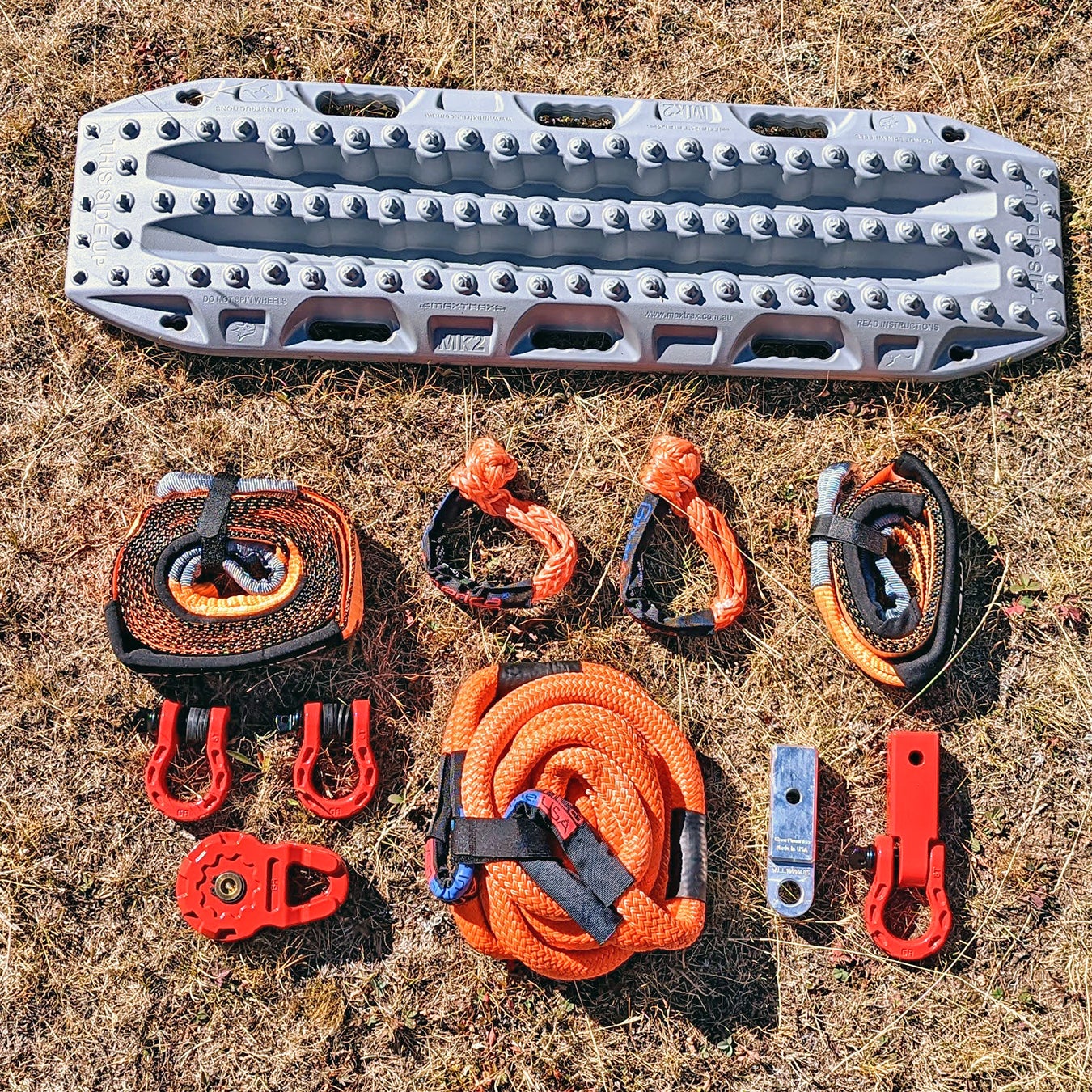The image is an overhead shot taken under very bright light, capturing a neatly arranged set of heavy-duty rescue and towing equipment laid out on a patch of dried, crispy brown grass. Center stage is a large, gray, plastic board with numerous dips, divots, and circular crevices, prominently labeled "this side up" on both ends, indicating its specific orientation for use, likely for carrying individuals during rescue missions. Below the board, in organized rows, are various pieces of high-visibility, bright orange safety equipment. These include coiled ropes with spliced loops, tightly coiled straps, and multiple metal attachments with safety screws, possibly used for pulleys or towing. The entire arrangement exudes a sense of preparedness and durability, suggesting that this equipment is designed to handle significant weight and pressure, potentially for scenarios such as mountain rescues via helicopter or vehicle towing.